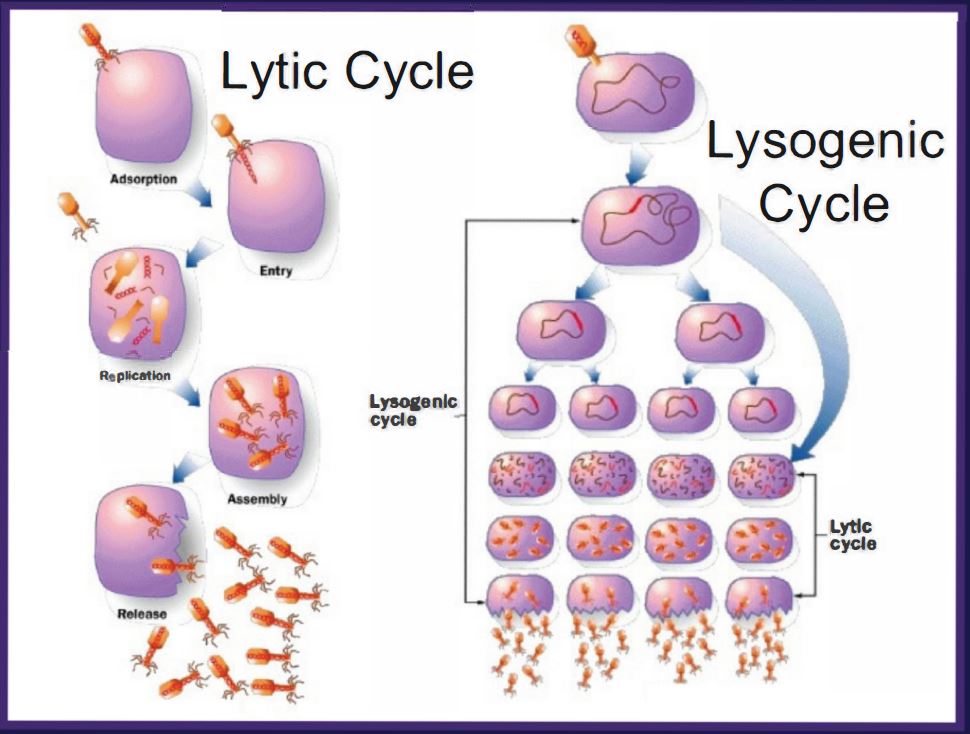The image is an informational graphic with a white background and a blue border, divided into two sections: the lytic cycle on the left and the lysogenic cycle on the right. Both sections contain multiple purple, rectangular-shaped blobs that represent cells. 

On the left side, under the heading "Lytic Cycle," the sequence starts with a single cell labeled "Adsorption," where an orange projection enters the cell. This is followed by stages labeled "Entry," "Replication," "Assembly," and finally, "Release," with blue arrows directing the flow from one stage to the next. As the stages progress, the contents within the cells resemble little bugs or particles. By the "Release" stage, these particles are released from the cell in large numbers.

On the right side, under the heading "Lysogenic Cycle," a different process is depicted. It starts with a single cell at the top, which then undergoes stages shown by arrows pointing downward. The contents appear to replicate more slowly and methodically, as one cell splits into two, and then each of those splits again, resulting in four cells. These stages indicate a more gradual increase in the number of particles compared to the explosive release seen in the lytic cycle. The overall structure and flow illustrate the contrasting mechanisms of viral replication in these two cycles.